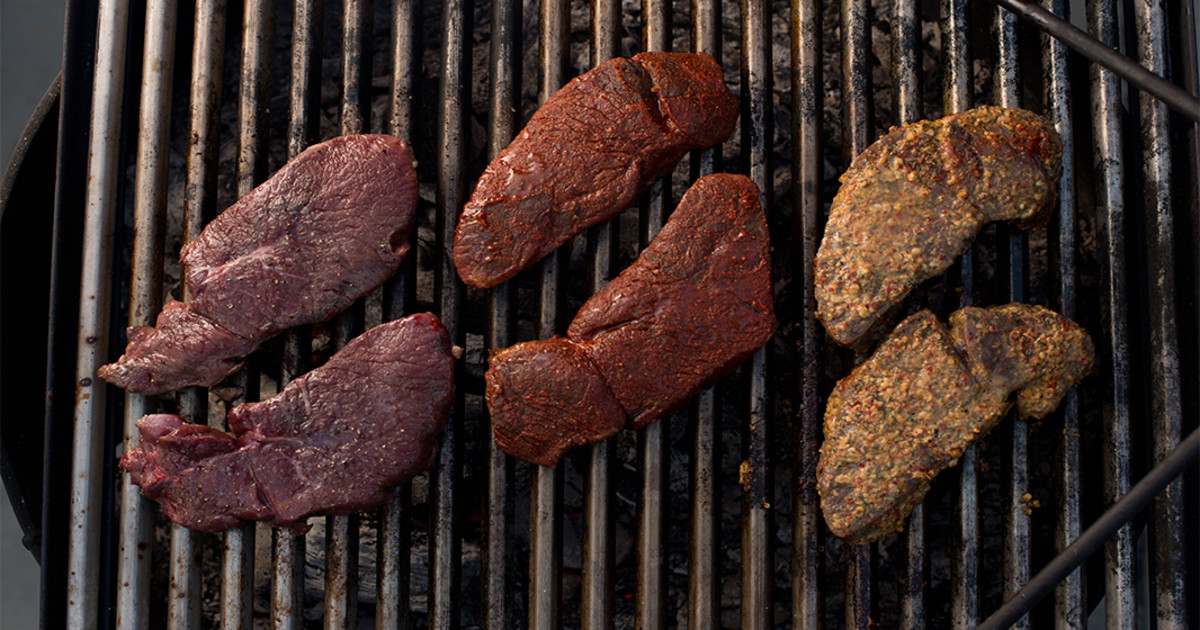The image portrays a top-angle view of an outdoor charcoal grill, likely taken by a food enthusiast. It appears to have been shot during the evening under artificial lighting, illuminating the scene. The grill is silvery grey with black shading, and there are clear signs of coal beneath the grill rods. Positioned neatly on the grill are six marinated steaks, each pair seasoned differently. The two steaks on the left side are pinkish with a simple salt and pepper seasoning. The middle steaks, more reddish-orange, are generously coated with red spices. The rightmost steaks exhibit a golden-brown hue, suggesting a lemon and herb marinade. The detailed arrangement and distinct marination of the steaks highlight careful preparation and culinary enthusiasm.